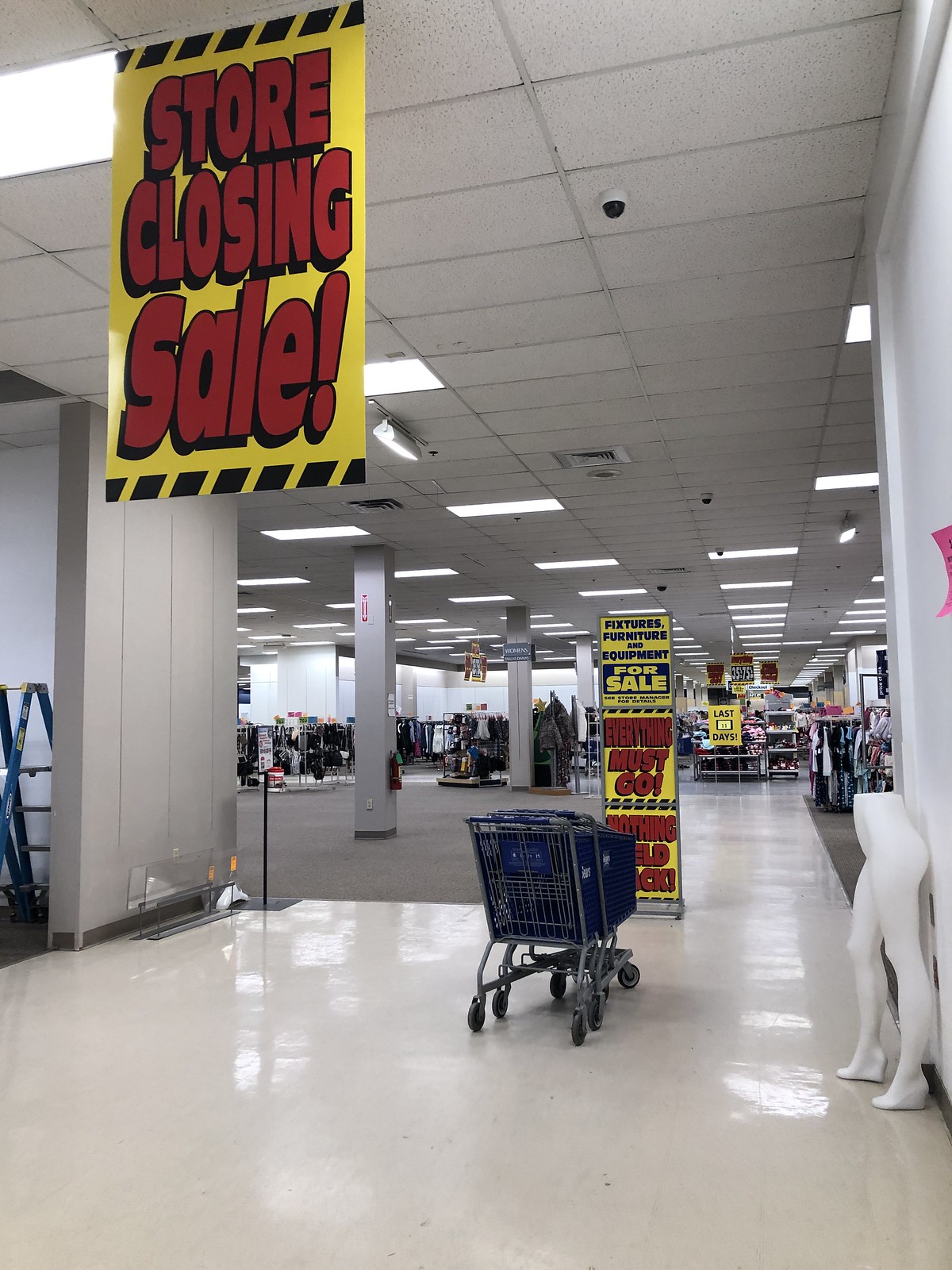This photograph captures the entrance to a large retail store amidst a "Store Closing Sale". The perspective is from just outside the entrance, where a short stack of shopping carts sits conspicuously in the middle of a gleaming, polished white linoleum floor. Leaning against the wall to the right is a stark white female mannequin, displayed from the waist down. Overhead, a prominent yellow sign with bold red letters announces the "Store Closing Sale". The interior view reveals a spacious layout, lined with square white columns that stretch up to a ceiling peppered with bright fluorescent lights set in tiles. More sale signs punctuate the scene, including one prominently placed on a stand right at the entrance. In the background, the store floor extends to reveal racks of clothing and shelves brimming with assorted merchandise, hinting at the final days of a once-thriving retail giant.